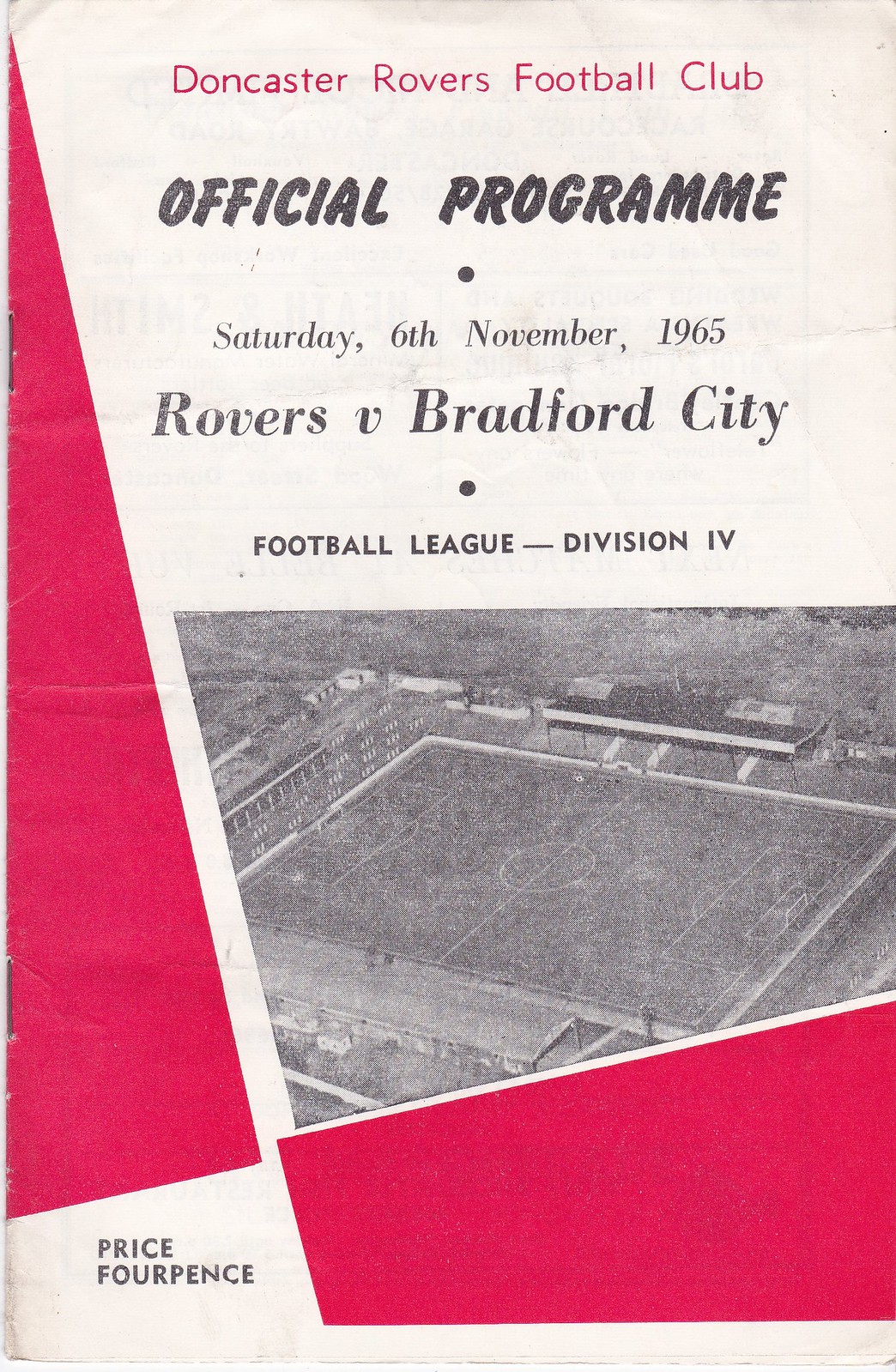This is the front page of an official program for the Doncaster Rovers Football Club, dated Saturday, 6th November 1965, for a Football League Division 4 match against Bradford City. The program is rectangular and beige with a distinctive layout, featuring a triangular red section on the left and a barely visible red rectangle diagonal to the bottom right corner. In the center, there is a striking black-and-white aerial photograph of a soccer stadium. The top of the page showcases the text "Doncaster Rovers Football Club" in bold red letters. Below it, in italicized black text resembling handwriting, is "Official Program" accompanied by the date "Saturday, 6th November 1965." Further down, it reads "Rovers vs. Bradford City," followed by "Football League Division IV." In the bottom left corner, the price is printed in black text: "Price Fourpence."